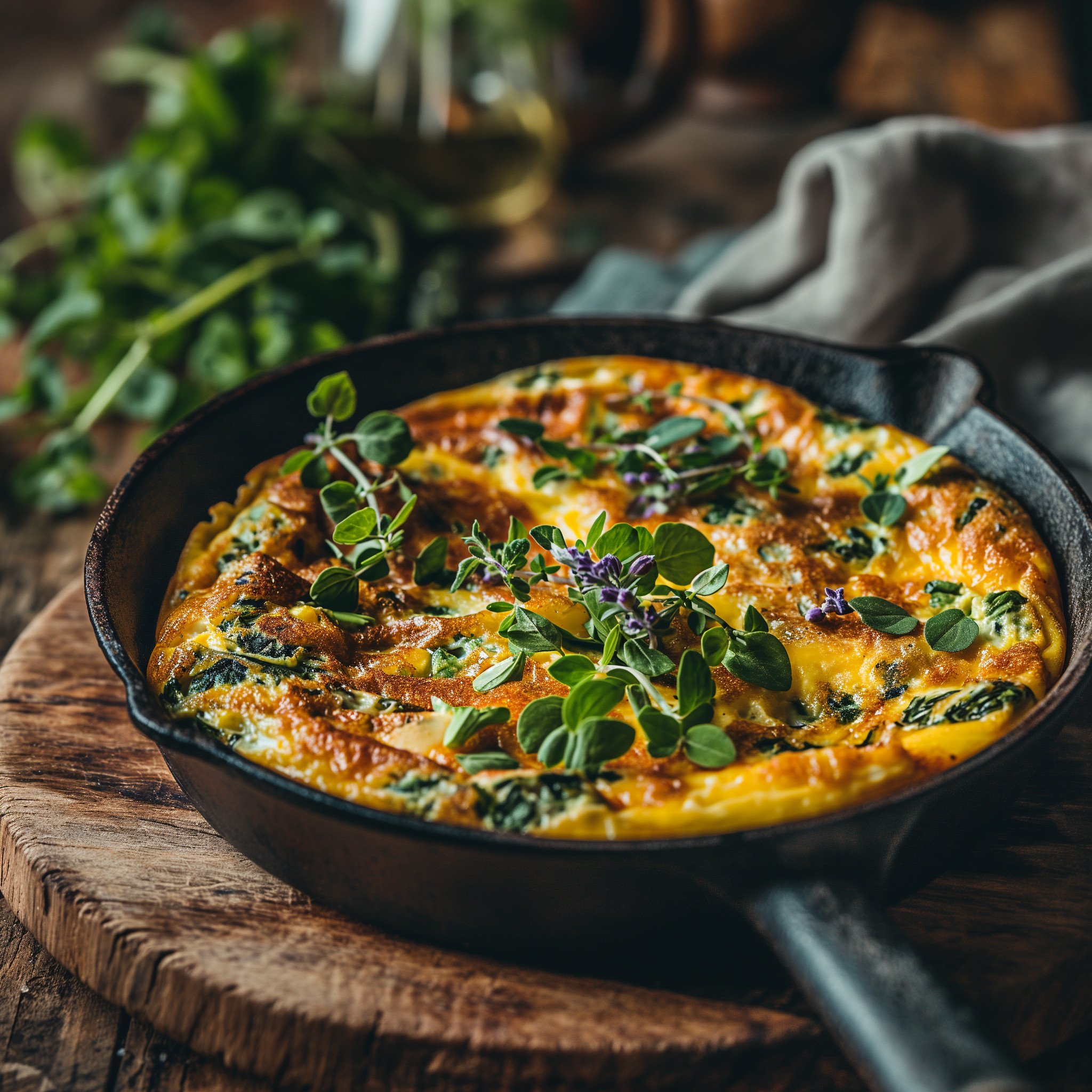This is a professionally composed, perfectly square photograph showcasing a round, deep, black cast iron skillet containing a fluffy, yellow-colored omelette, souffle, or possibly a thick pizza. The dish is garnished with green herbs, including likely spinach and basil, along with some burnt brown spots on the surface. The skillet has a handle protruding from the bottom right and is set upon a round wooden surface resembling a tree stump or cutting board. In the blurry background, the upper left features some greenery which appears to be the same as the herbs garnishing the dish, while the lower right contains what appears to be a gray towel. The impeccable lighting and shallow depth of field indicate this image was taken with professional equipment, enhancing the dish’s vibrant colors and textures.